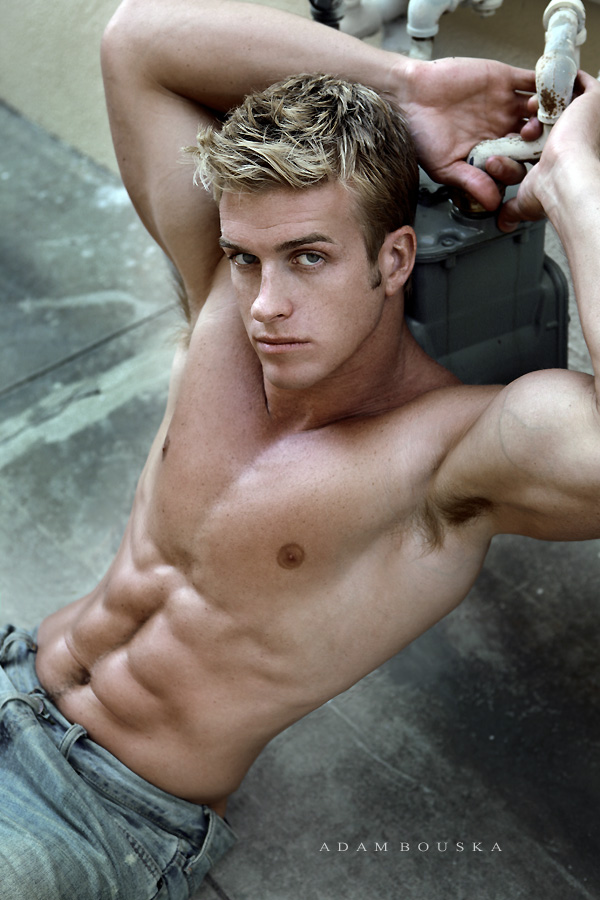In this striking photograph, a shirtless man is seated on a concrete floor, dressed in a pair of blue jeans. Positioned centrally within the frame, he gazes directly up at the camera with an intense, thoughtful expression. His hand grips a metal pipe situated behind him, adding an element of raw, industrial ambiance to the composition. The ground surface features various shades of gray and brown, contributing to the gritty urban aesthetic. The artist's name, Adam Buska, is inscribed at the bottom of the image, suggesting the work of a professional photographer. The setting remains ambiguous, suggesting it could be either an indoor studio or an outdoor urban environment. The overall color palette—gray, tan, white, brown, and yellow—enhances the rugged, natural feel of the scene, emphasizing the raw vulnerability of the model in this evocative portrait.